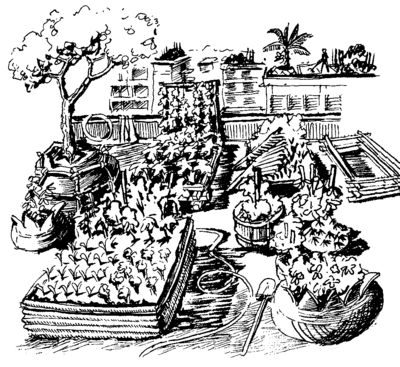This detailed black and white etching appears to depict a bustling farmer's market scene. At the forefront, there is a large square box brimming with vegetables, its perimeter lined with the fresh produce. Adjacent to this box on the right side, there is a basket filled with wheat or hay, accompanied by four smaller baskets. A hose trails up to the large vegetable box, while a shovel lies nearby. To the left of the vegetable box stands a tree and a planter, with a smaller bush or tree also housed in a planter beside it. Directly behind the vegetable box, a vine descends towards the base of another garden plot. To the right, a rectangular garden, currently vacant, is positioned next to a stack of vegetables or wheat. In the distant background, there are outlines of additional market stalls, trees, and a man tilling the soil, contributing to the lively yet serene market atmosphere.